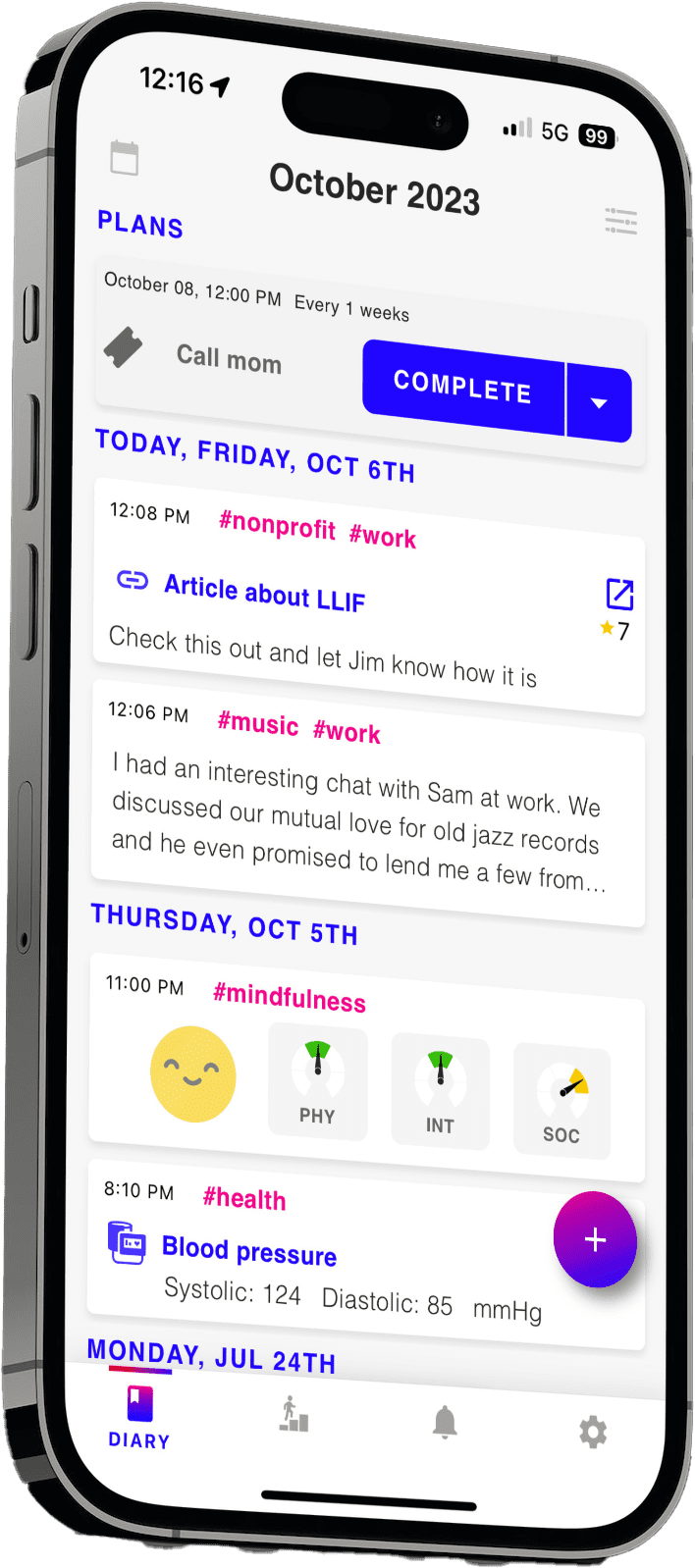A screenshot captures a smartphone's interface showcasing an organizational application. At the top center, the display reads "October 2023," indicating the current month. Below, a series of scheduled plans and tasks is listed:

1. "October 8th, 12 p.m. - Every one week: Call Mom" marked with "Complete."
2. "Today, Friday, October 6th - Article about LLIF."
3. "Thursday, October 5th - Mindfulness and Health."

The interface includes additional descriptions and details pertaining to each task.